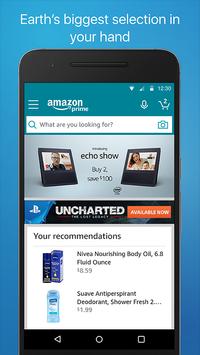The image is an advertisement for Amazon, featuring a blue background with a prominent mobile phone displaying the Amazon website. The banner above the smartphone reads in white letters, "Earth's biggest selection in your hand," emphasizing Amazon’s vast product availability. 

On the phone screen, the Amazon interface is visible, indicating that the user has two items in their shopping cart, as shown by the cart icon in the top right corner. The interface includes a microphone icon near the Amazon Prime section, suggesting that voice recognition is supported. Below the microphone icon, there is a search dialog box that allows users to type in queries or use a camera feature to search by image.

Further down the screen, there is an advertisement for the Echo Show, promoting a deal: "Buy two, save $100." Below this banner, several personalized product recommendations are displayed, including Nivea Nourishing Body Oil and an antiperspirant product. The overall composition of the image conveys the ease and variety of shopping on Amazon, accessible directly from your mobile device.